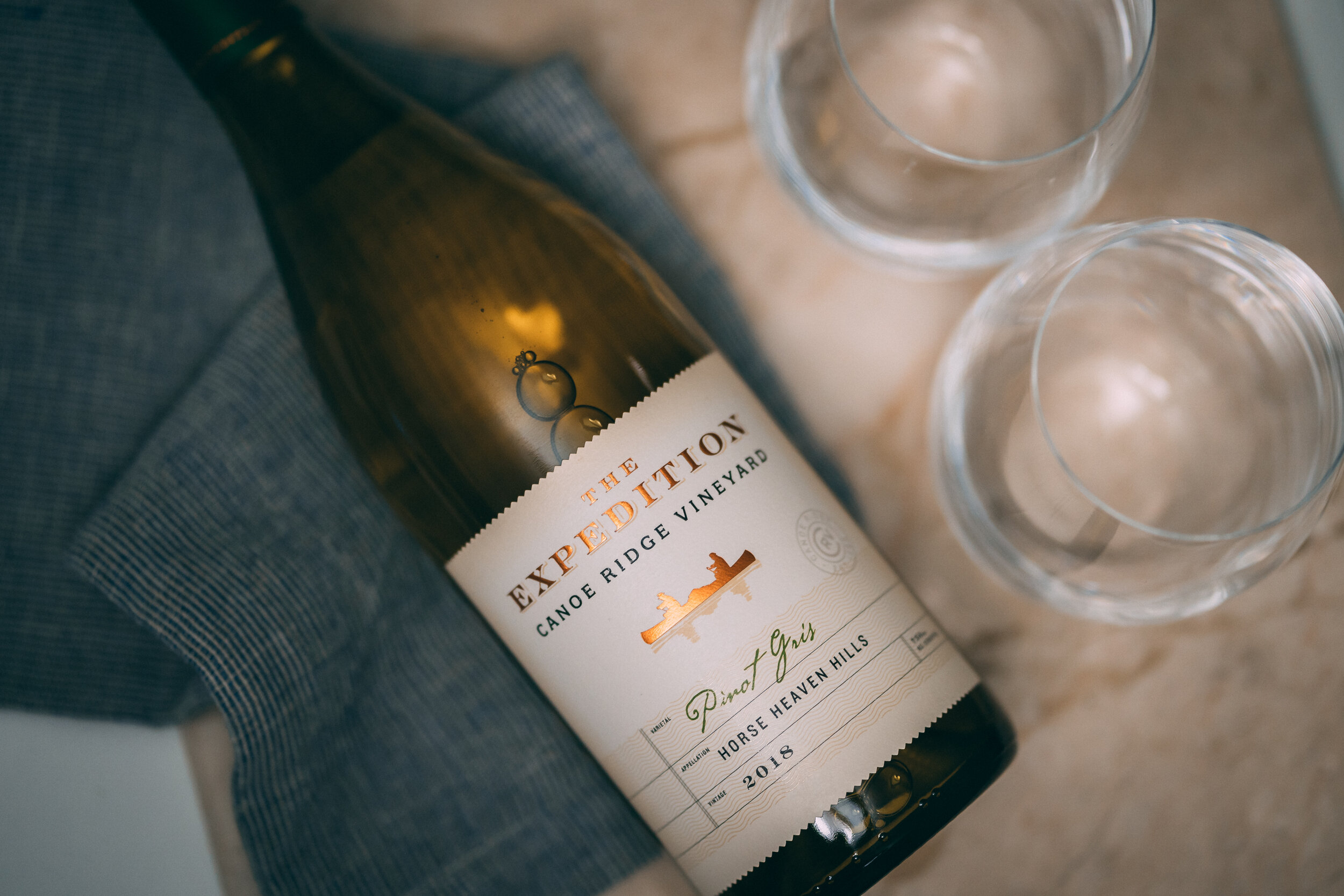The image features a detailed and well-composed photograph taken directly from above, capturing a green bottle of "The Expedition" wine from Canoe Ridge Vineyards. The bottle, which bears a white label with gold and green accents, showcases the brand name in gold, with an elegantly depicted gold canoe and two paddlers. Below this imagery, the label reads "Pinot Grigio," "Horse Heaven Hills," and "2018" in green text. The bottle is lying flat on its side atop a folded, denim-like blue cloth on a finely veined marble countertop, predominantly white with gold-brown streaks. Two stemless wine glasses are positioned in the upper right, appearing slightly above and to the side of the bottle, seemingly empty to almost clear, resting on the same marble surface. This staging highlights the bottle's label and adds a sense of casual elegance to the overall composition.